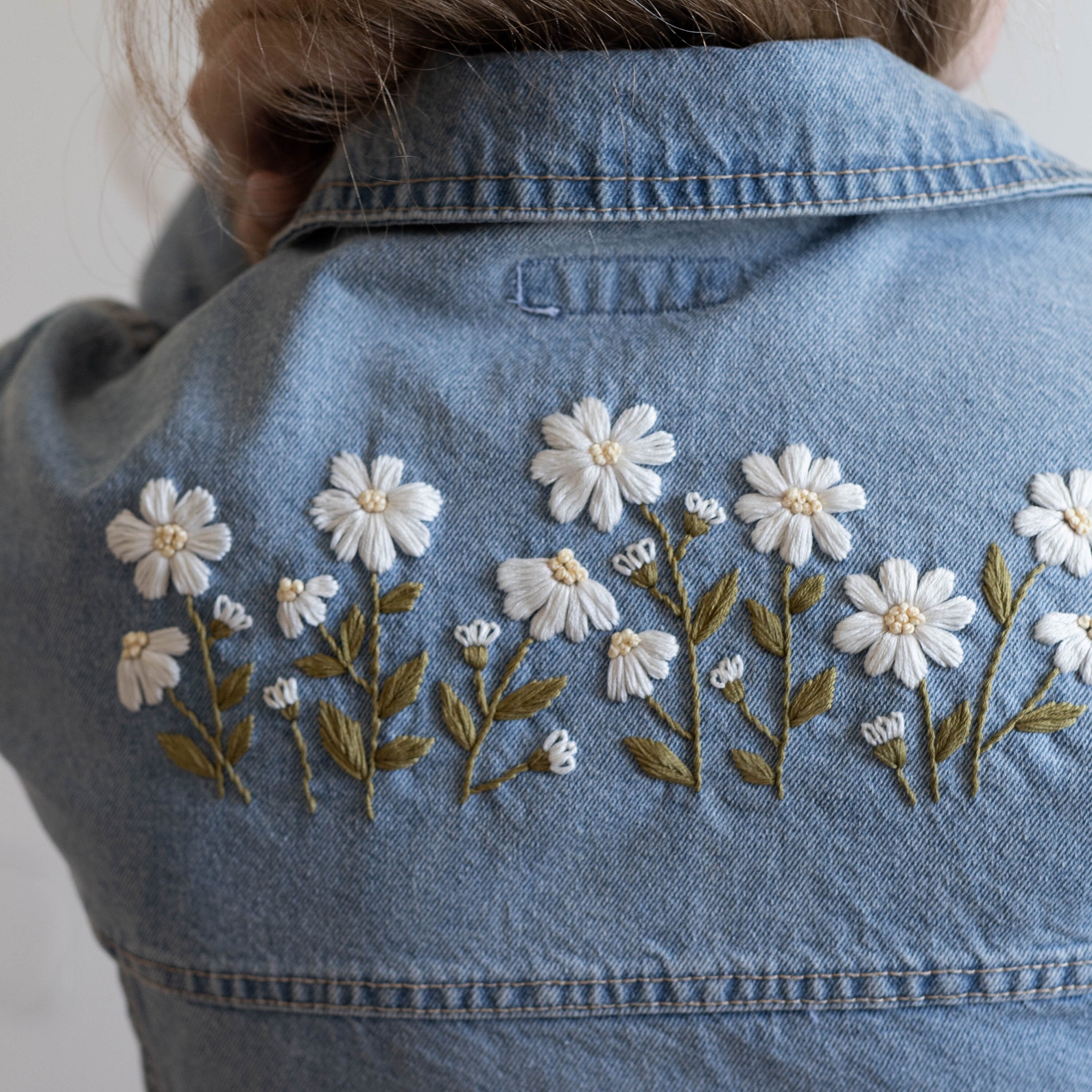The image is a square photograph featuring a light blue jean jacket against an off-white background, showcasing intricate embroidery on the back. You can see the top of the person's head with brownish-blonde hair tucked in, and their hand is up on the collar, revealing the long sleeve of the jacket. The embroidered detail consists of a line of flowers across the upper back and shoulders. The flowers, which resemble daisies, have green stems and leaves. The petals are white with yellow centers, and each full flower has eight petals. Additionally, there are partially opened flowers displaying half their petals, as well as small buds, depicted as three white loops at the end of a stem. The person wearing the jacket appears to be a Caucasian female, and the image offers a detailed view of both the embroidery and her casual pose.